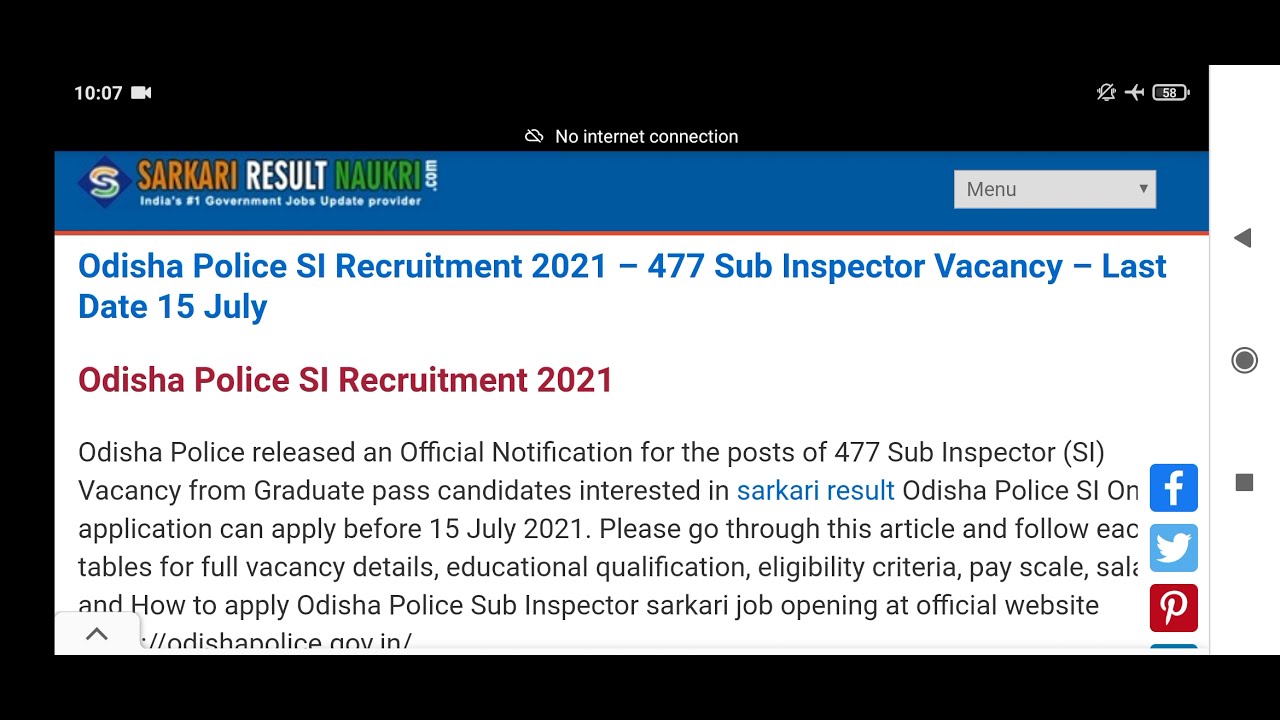The image displays a job posting on the screen of someone's phone. At the top, a blue bar reads "Sarkari Results Now Creep.com," stating that it is India's number one government jobs update provider. Below, it announces "Odisha Police SI Recruitment 2021 - 477 Sub-Inspector Vacancy" with the application deadline as July 15th, 2021. The image also features details about the recruitment, specifying Odisha Police's official notification for 477 sub-inspector posts available for graduate pass candidates. The article invites applicants to read further for full details on vacancy specifics, educational qualifications, eligibility criteria, pay scale, salary, and application procedures through the official website. Additional elements displayed on the phone include the date, time, no internet connection icon, battery status, airplane mode icon, and social media icons for Facebook, Twitter, and Pinterest.